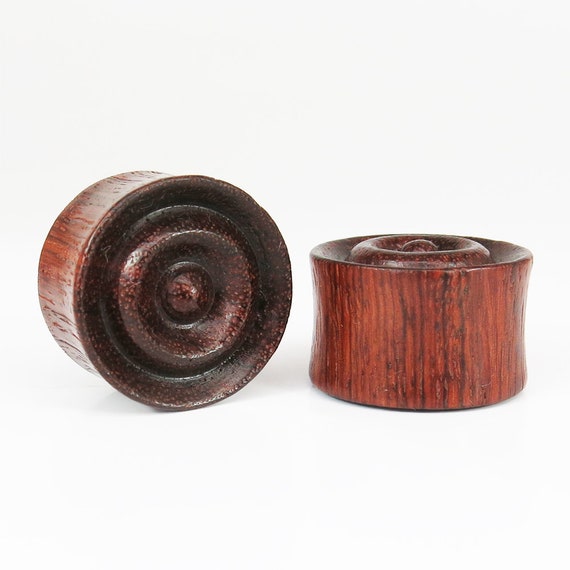The photograph features two small wooden objects set against a clean, white background. Each piece appears circular or cylindrical, resembling halves of a cylinder. The outer edges of these objects have a dark brown or maroon hue adorned with black stripes, giving a visually rich wooden texture. The wood's exterior on both pieces seems slightly compressed towards the center, suggesting they might have been pinched or squeezed. The tops of the objects showcase intricate, spiral-like channels, akin to the decorative grooves found on chess pieces, with a dark, grainy, and shiny finish. Both pieces are positioned distinctly: one lies on its side, suggesting it could roll, while the other stands upright, as if reaching towards the sky. These objects, though their exact purpose is unclear, could serve as paperweights or decorative artifacts, with their detailed design and small stature hinting at a role in finer woodworking or furniture design.